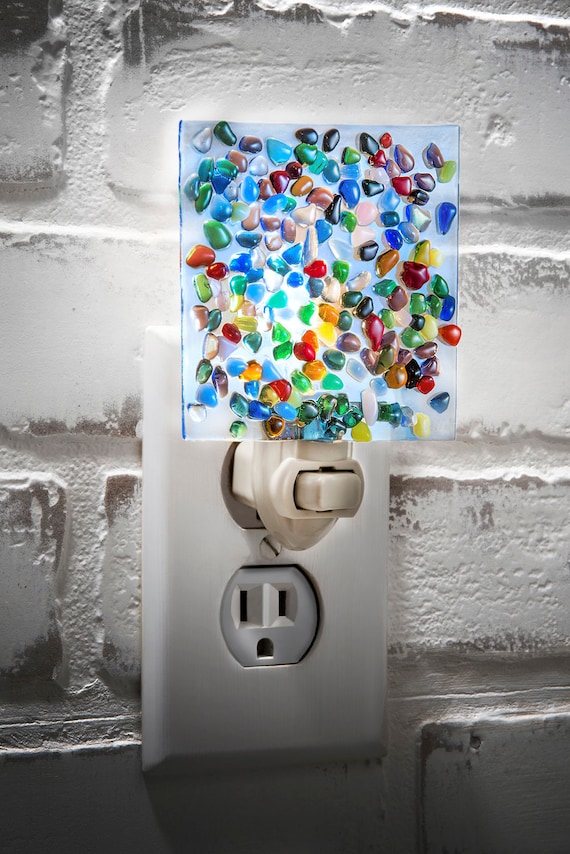This photograph showcases an inventive nightlight installed on a white-painted brick wall. Plugged into a white electrical outlet, the nightlight itself is an off-white or ivory color and features an on-off switch at its base. At the top, where the light bulb is likely installed, a creative touch has been added: a roughly 4-inch by 4-inch piece of blue plastic or glass. This square is intricately adorned with around 80 to 100 tiny, multicolored stones, including hues of blue, brown, red, and yellow. These stones not only soften the light emitted by the nightlight but also create a visually striking effect that adds both subtle illumination and aesthetic charm to the room.